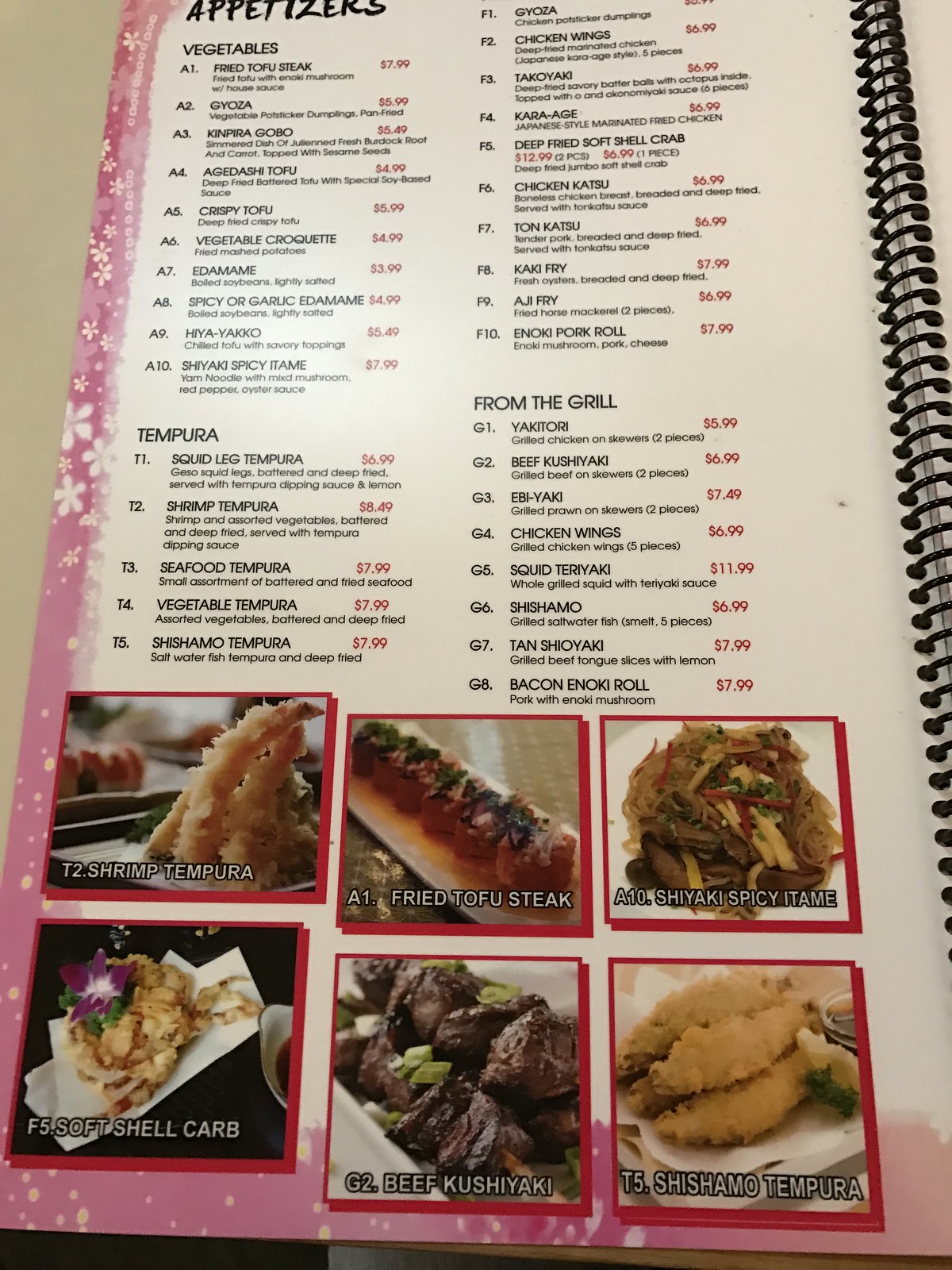This photograph showcases a partial view of a restaurant menu, cut off at the top, truncating the word "Appetizers" slightly. A black spiral binding is visible along the right edge, particularly prominent towards the top. The bottom section of the menu features six labeled photographs:

- T2: Shrimp Tempura
- A1: Fried Tofu Steak
- A10: Shiitake Spicy Atami
- F5: Soft Shell Crab
- G2: Beef Kushiyaki
- T5: Shishamo Tempura

Above these photographs, the menu is organized into sections labeled "Appetizers," "Vegetables," "Tempura," and "From the Grill." Each item is listed with a corresponding alphanumeric code, a name, a description, and a price highlighted in red font, contrasting with the black text used for the rest of the menu.

The menu has a distinctive pink border adorned with animated floral graphics and scattered dots as you move further down the page. Each food photograph at the bottom is enclosed in an embossed-looking red frame, adding a touch of elegance to the presentation. The background of the menu is predominantly white, which accentuates the vivid pink border and floral motifs.